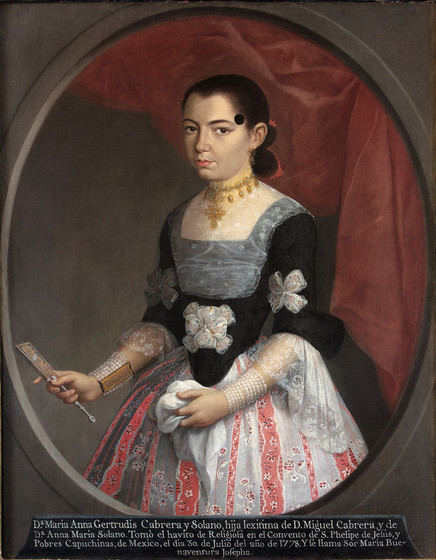This painting is a captivating portrait featuring a woman set against a brown rectangular background, encased in a similarly brown vertical oval frame. The subject, a distinguished woman, dons a striking dress with a black top outlined in grey around the chest and a skirt featuring light grey with vertical red stripes adorned with a white flower pattern. She has silver bows on each arm and one on the abdomen, complementing the strings of pearls adorning her wrists. In her right hand, she holds a closed silver fan, while her left hand clutches a bunched-up piece of her skirt. The woman wears an ornate golden necklace draped around her neck and chest. She has dark brown hair arranged in a bun at the back and a prominent black beauty mark on the left side of her face. A crumpled red curtain, descending at a sharp angle from left to right, forms the background. At the bottom, a black frame contains a caption in Spanish, stating: "Di Maria Anna Gertrudis Cabrera y Solana, hija lexerima de Miguel Cabrera y de Diana Maria Solana, tomo el habito de religiosa en el convento de San Felipe de Jesus y Pobres Capuchinas de Mexico del sin tercero de Julio del año de 1778 y se llama Sor Maria Buenaventura Josefina."